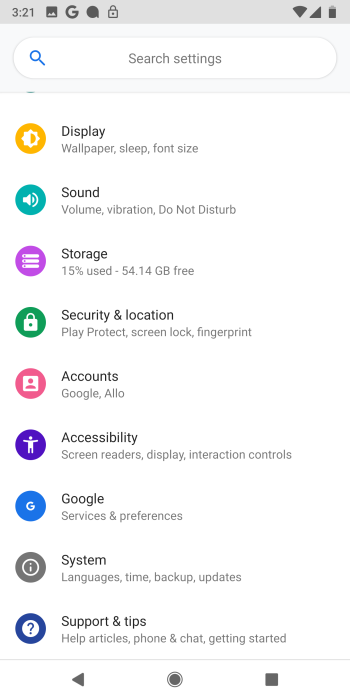This image appears to be a screenshot of a mobile phone's settings menu. At the very top, the regular status bar is visible, displaying essential information such as the time (3:21), a small Google icon, a lock icon, network usage, and battery status. Below the status bar is a search box with a blue magnifying glass icon, containing the text "Search settings" in light gray.

Proceeding further down, the settings menu is divided into several sections with corresponding icons and options:

1. **Display** (orange icon) - Options include Wallpaper, Sleep, and Font size.
2. **Sound** (green icon) - Options include Volume, Vibration, and Do Not Disturb.
3. **Storage** (purple icon) - Displays usage information, noting that 15% of 54.14 GB has been used.
4. **Security & Location** (green icon) - Options include Play Protect, Screen Lock, and Fingerprint.
5. **Accounts** (pink icon) - Options include Google and Allo.
6. **Accessibility** (purple icon) - Options include Screen Readers, Display, and Interaction Controls.
7. **Google Services & Preferences** (blue icon).
8. **System** (gray icon) - Options include Language, Time, Backup, and Updates.
9. **Support & Tips** (blue icon) - Options include Help Articles, Phone and Chat, and Getting Started.

At the very bottom of the screen, three navigation icons are present: a leftward arrow for Back, a circle for Home, and a square for Recent Apps.